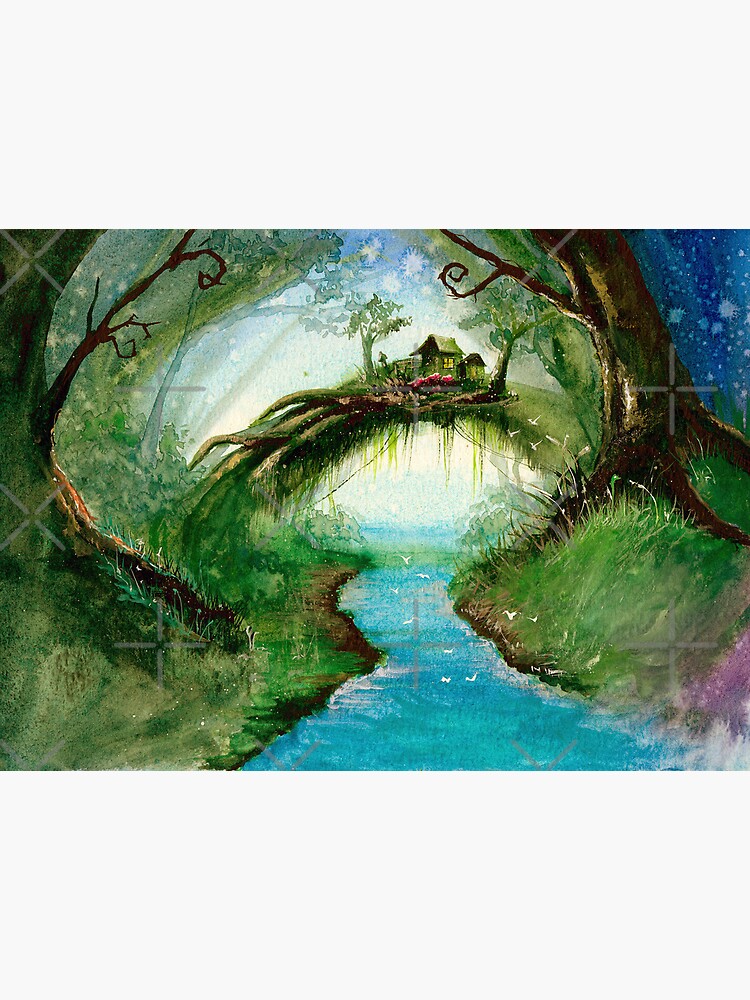This rectangular fantasy illustration, measuring approximately 6 inches tall by 4 inches wide, depicts an enchanting, otherworldly scene. The detailed watercolor painting is framed by light gray headers and footers at the top and bottom of the image.

The centerpiece features a diminutive house perched precariously on intertwined tree roots that form an arched bridge. This bridge stretches gracefully over a small blue stream that meanders through the center of the scene. The stream's edges, tinged with brown earth, transition smoothly into verdant grassy hills that flank both sides of the water.

Towering tree trunks mark the boundaries of the illustration on the far left and right, with lush green bushes and shrubs adding to the forest ambiance. The house atop the roots, with its tiny garden, exudes a whimsical charm, reinforcing the fantastical nature of the illustration. The colors used, predominantly greens and blues, contribute to the dreamlike quality, making it reminiscent of a scene from a fantasy book.